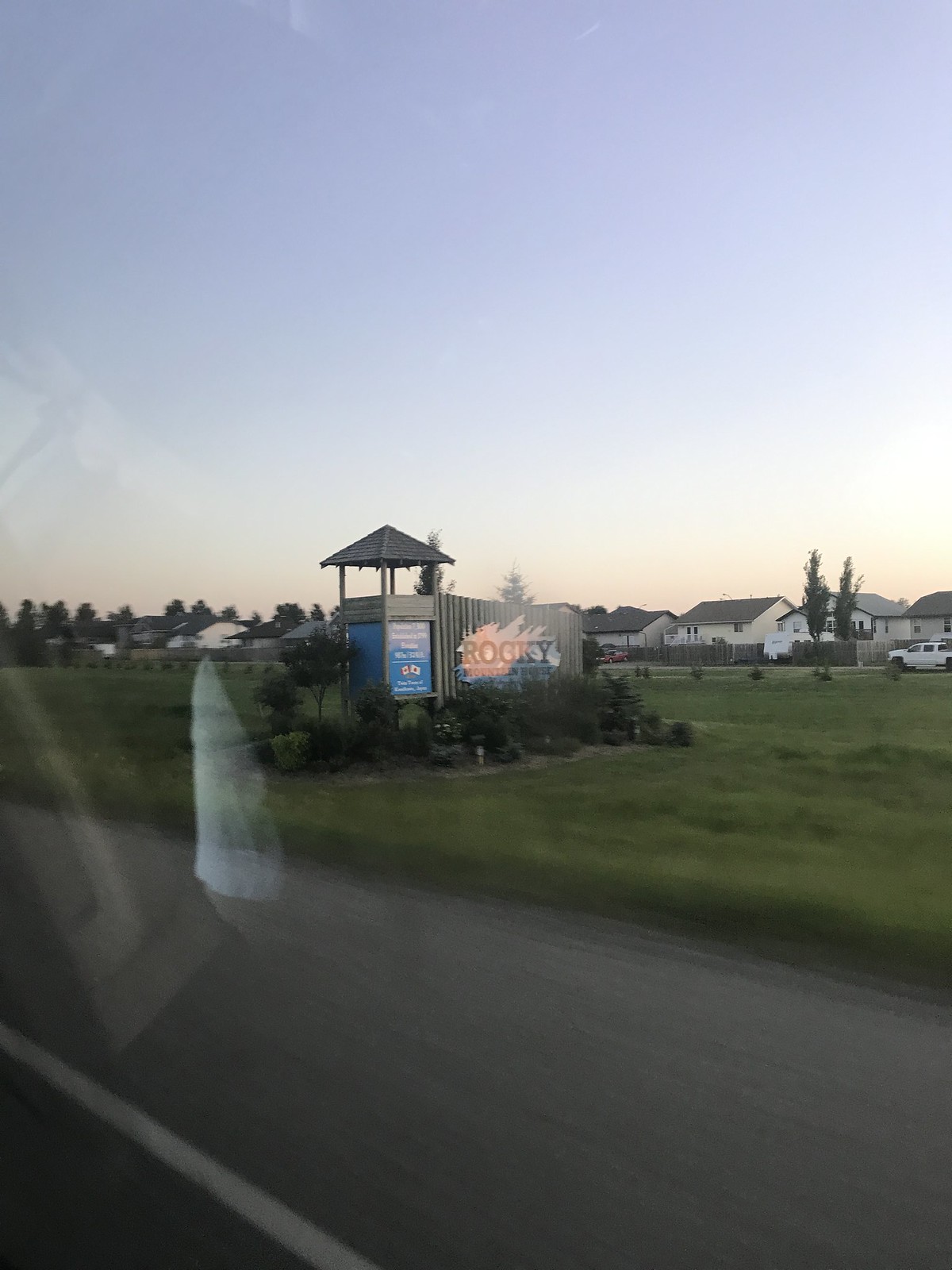This image captures a scene from inside a moving car, evident from the blurred details and the reflection of a person's sleeve on the car's window. Taken through the rolled-up window, the main focus is a large wooden sign featuring the text "Rocky Mountain House," partially obscured below, supported by slatted gray posts. The sign is topped with a small, attached wooden tower that resembles a gazebo with a three-dimensional, triangular gray roof. Adjacent to the sign, there is a booth with a canopy-like roof, adorned with both the Canadian and Japanese flags. Surrounding the sign are lush green bushes and a meadow of grass. To the left, a roadway with a white line is visible, indicating the car’s path. In the background, a quiet neighborhood stretches out under a clear blue sky, suggesting the setting sun.